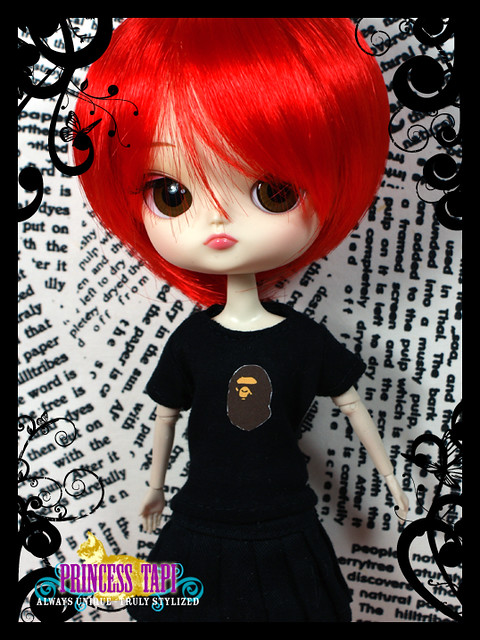The image is a detailed color photograph of a distinctive doll with a dramatic appearance. The doll has a notably large head, vibrant red hair styled in a bob cut, and expressive brown eyes. It features a fair complexion, a small, delicate nose, and a petite mouth. The doll's slim neck supports a contrastingly large head, giving it a whimsical look. It is dressed in a black t-shirt and a matching black skirt. The black t-shirt bears a brown and yellow oval-shaped design, possibly depicting a character or an abstract pattern.

The doll's thin, articulated arms are positioned at its sides, with joints visible at both the elbows and wrists. The setting behind the doll consists of numerous overlapping sheets of paper densely printed with black text in various orientations, creating a chaotic yet intriguing background.

Framing the image is a black border adorned with intricate scroll designs and plant-like curlicues, along with butterflies and vines enhancing the whimsical theme. In the lower left-hand corner, a pink, yellow, and blue logo reads "Princess TAPI" in bold letters, with the tagline "Always Unique, Truly Stylized" written below in white text. This captivating and eclectic photograph captures the unique charm of the doll, juxtaposed against a richly textured and patterned backdrop.